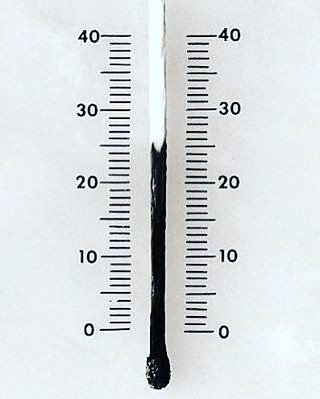The image depicts a creative yet unpolished drawing of a thermometer. The thermometer is fashioned from two pieces of paper, each labeled with a scale ranging from 0 to 40 degrees. The scales appear to have been printed from a computer, given their precise, machine-generated lines and lack of hand-drawn characteristics. These two pieces of paper are placed side-by-side with a slight gap between them. At the bottom of the scales, underneath the zero markers, the artist has sketched the bulb of a thermometer. The bulb and the section of the thermometer up to the 25-26 degree mark are filled in with black coloring. The coloring, however, is inconsistent and leaves patches of white visible through the black. The edges of the cutout on the right side are notably rough and jagged, displaying visible tracing marks indicative of a hasty or careless cutting job. The entire arrangement is placed on a white background, which blends with the white paper, potentially enhancing the illusion of a thermometer at first glance. The thermometer drawing fails to extend beyond the 40-degree mark.